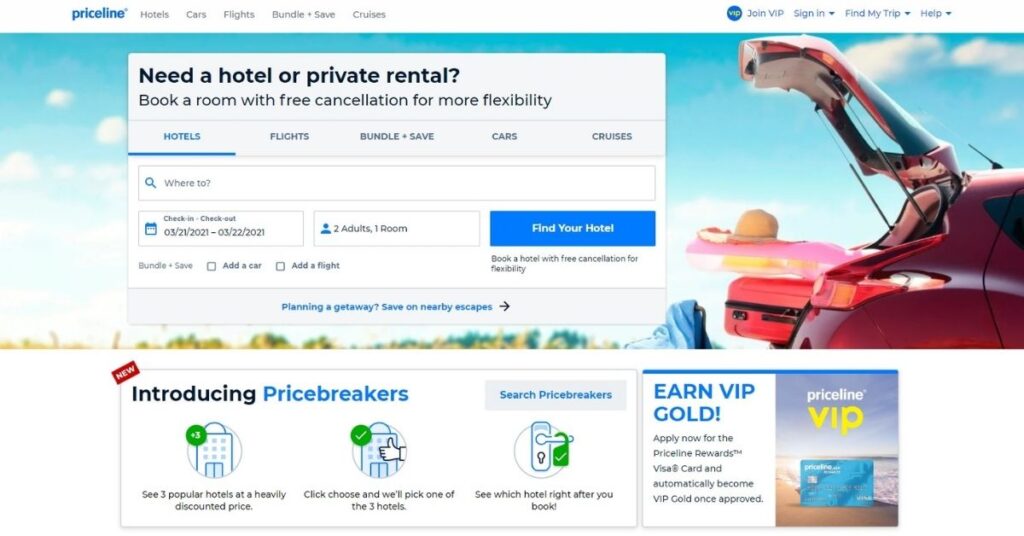The image features a vibrant blue background with "Priceline" prominently displayed in blue text at the top. Below that, several headers are listed, each followed by down arrows indicating dropdown menus. Positioned centrally is a striking photograph showcasing a red car with its trunk open, set against a picturesque blue sky filled with white, fluffy clouds. In the distant background, a little brown, round object is visible.

To the right of the image, a large white box contains bold text reading, "Need a Hotel or Private Rental? Book a room with free cancellation for more flexibility." Beneath this promotional message is a series of navigational links: "Hotels" underlined in blue, "Flights," "Bundle and Save," "Cars," and "Cruises."

A search box equipped with a magnifying glass icon enables users to input their destination under the field labeled "Where To." Adjacent to this are fields for selecting check-in and check-out dates, alongside an option for specifying occupancy, defaulting to "two adults in one room." Below, a prominent blue button labeled "Find Your Hotel" facilitates the search process. Additional options to "Add a Car" or "Add a Flight" are also presented.

The lower section of the image features several promotional elements. One white box highlights the text "New," followed by a red box introducing "Price Breakers." This section showcases three popular hotels offered at frequently discounted prices. A call-to-action, "Choose," encourages users to select one of the three hotels, with the final selection revealed after booking.

Another box with a thick blue top border introduces "Earned VIP Gold" under the "Priceline VIP" program, featuring an image of a credit card, likely illustrating an exclusive offer or loyalty reward.